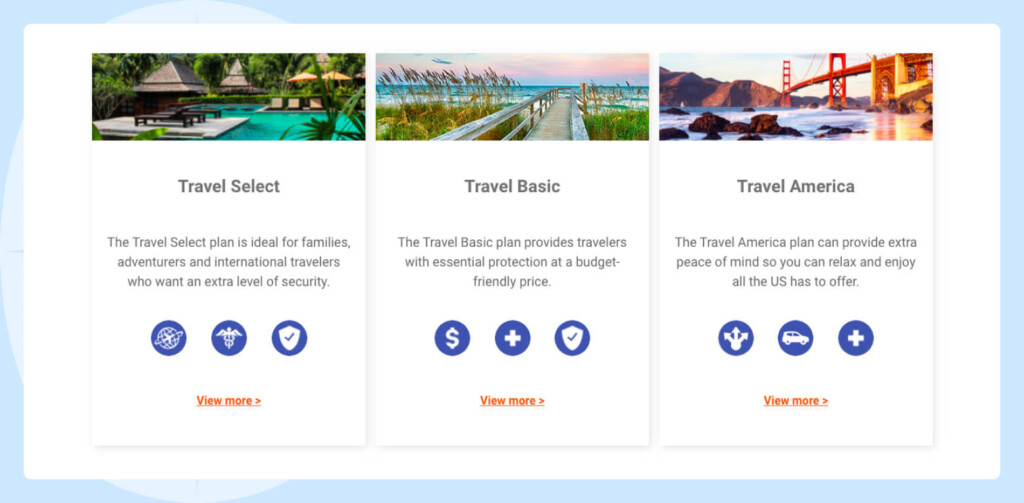The image features a travel-themed webpage adorned with a blue border encasing a predominantly white background. Spanning the top of the page are three distinct photographs.

The first image on the left depicts an exotic outdoor scene with a distinct Asian influence. Central to this scene is a triangular hut perched on a platform above a serene body of water, evoking a sense of tranquility and escape.

The middle photograph portrays a breathtaking outdoor view at sunset. A narrow footbridge with railings on either side, constructed of wooden slats, stretches towards the water, capturing the fading light of the sun as it sinks beyond the horizon.

The third image on the right offers a scenic vista of a bridge set against a backdrop of majestic mountains and a flowing body of water, combining natural beauty with structural elegance.

Below each photograph are captions describing different travel plans:

- Beneath the Asian-themed scene, the caption reads, "Travel Select." It describes the Travel Select plan as being perfect for families, adventurers, and international travelers seeking added security.

- Underneath the sunset scene, the caption states, "Travel Basic." This text highlights the Travel Basic plan as providing essential protection for travelers at an affordable price.

- Below the bridge and mountain photograph, the caption proclaims, "Travel America." It emphasizes that the Travel America plan offers additional peace of mind, allowing travelers to fully relax and enjoy all that the United States has to offer.